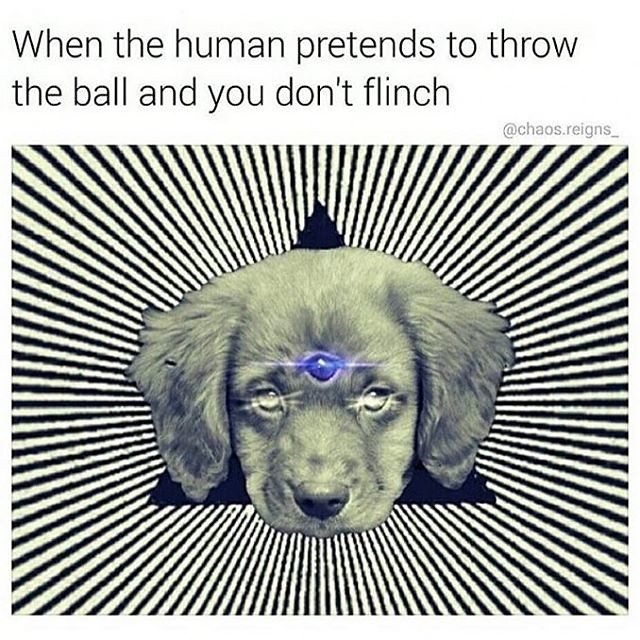The image is a computer-generated artwork featuring a black and white puppy with floppy ears, placed centrally over a black triangle. The background consists of intricate black lines radiating outward in various directions on a dull white backdrop. The puppy's eyes appear illuminated, emitting light that gives them a laser-like appearance. Additionally, the puppy has a blue jeweled gem embedded in the center of its forehead, also glowing faintly. Above the main image, the text reads, "when the human pretends to throw the ball and you don't flinch," drawing attention to the puppy's composed expression amidst the visually striking elements. The overall design evokes an otherworldly, Illuminati-like aesthetic with its geometric shapes and light effects, creating a intriguingly surreal portrait of the dog.